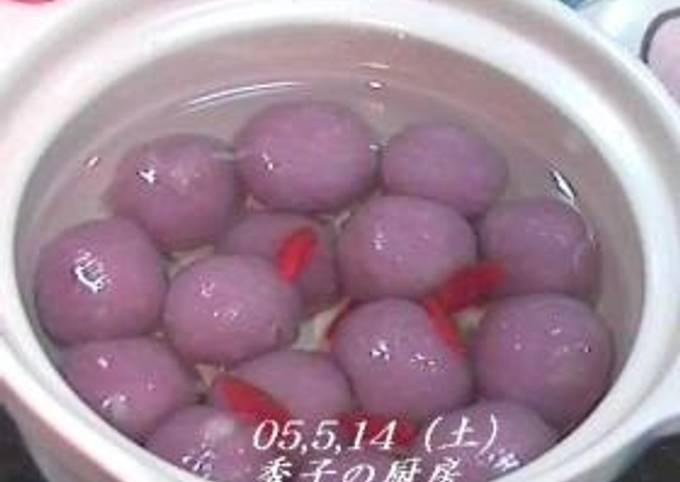This photograph features a white bowl containing round, purple items that resemble small lemons, submerged in water. The bowl, filled with approximately twenty of these violet spheres, also contains some red-colored stems among them. At the bottom center of the image, there are numbers written in white—05, 5, 14—along with some foreign text that appears to be either Chinese or Japanese.